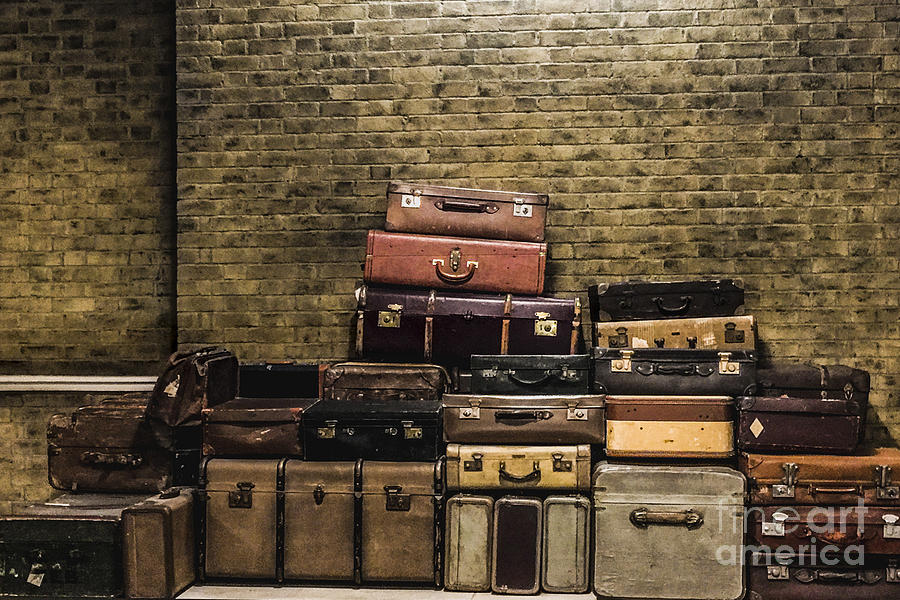In this image, a neatly stacked collection of vintage luggage rests in front of a large, dark brown brick wall that features black splotches and lighter brown hues. The assortment includes both suitcases and trunks, characterized by their hard-shell exteriors, which enable them to be securely piled on top of each other. The bottom row on the left consists of light brown suitcases, transitioning to dirtied white ones, and then darker brown ones on the right. A striking yellow suitcase stands prominently in the center, with its handle facing forward, flanked by darker brown suitcases on both sides. Above the yellow suitcase, a dark brown suitcase is visible, with two rose-colored suitcases stacked even higher. The collection features a variety of colors, sizes, and brands, with many pieces equipped with traditional side locks. This meticulously organized display of antique luggage, which includes small black suitcases, larger black suitcases, tan suitcases, a brownish-red suitcase, and trunks in shades of gray and tan, reaches approximately three-quarters of the way up the wall.